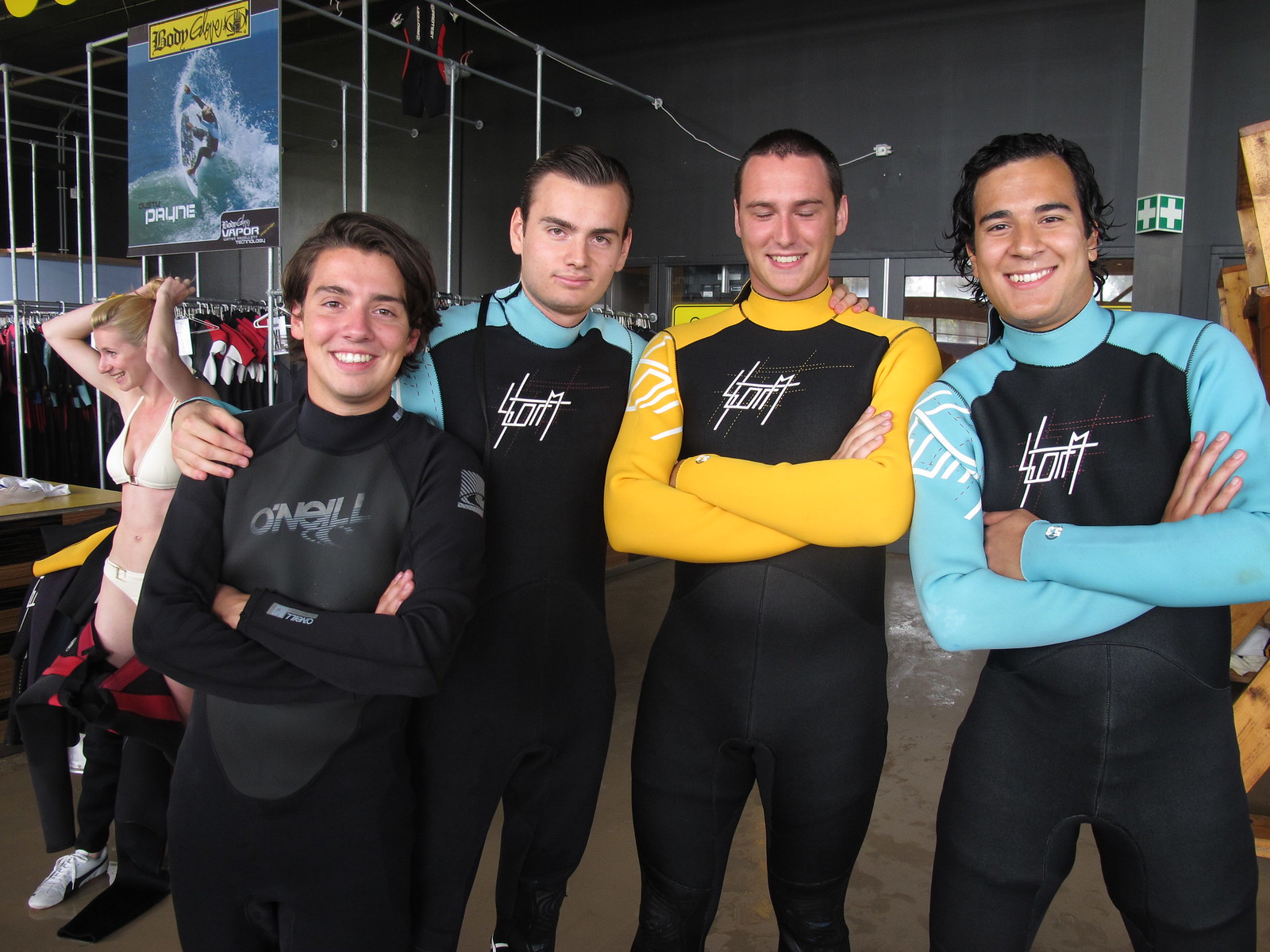This is a detailed color photograph capturing four young men posing together in what appears to be a retail shop, evident by the racks of wetsuits and an advertisement for Body Glove in the background. They are all wearing wetsuits, with three of them donning the same brand called "STORM" and featuring a jagged T-S shaped logo. 

From left to right:
- The first man is in a black wetsuit with gray accents, branded by O'Neill. He appears to be the youngest, around 19 years old.
- The second man is wearing a black wetsuit with turquoise trim, about 25-28 years old, and smiling directly at the camera.
- The third man, also around 25-28 years old, has his eyes closed and a big smile on his face. His wetsuit features black and yellow colors with the "STORM" brand.
- The fourth man, similarly aged, is smiling widely wearing a black wetsuit with turquoise accents and the "STORM" logo.

To the far left of the group, there is a woman in a bikini, tying her hair back and smiling as she prepares to put on her wetsuit.